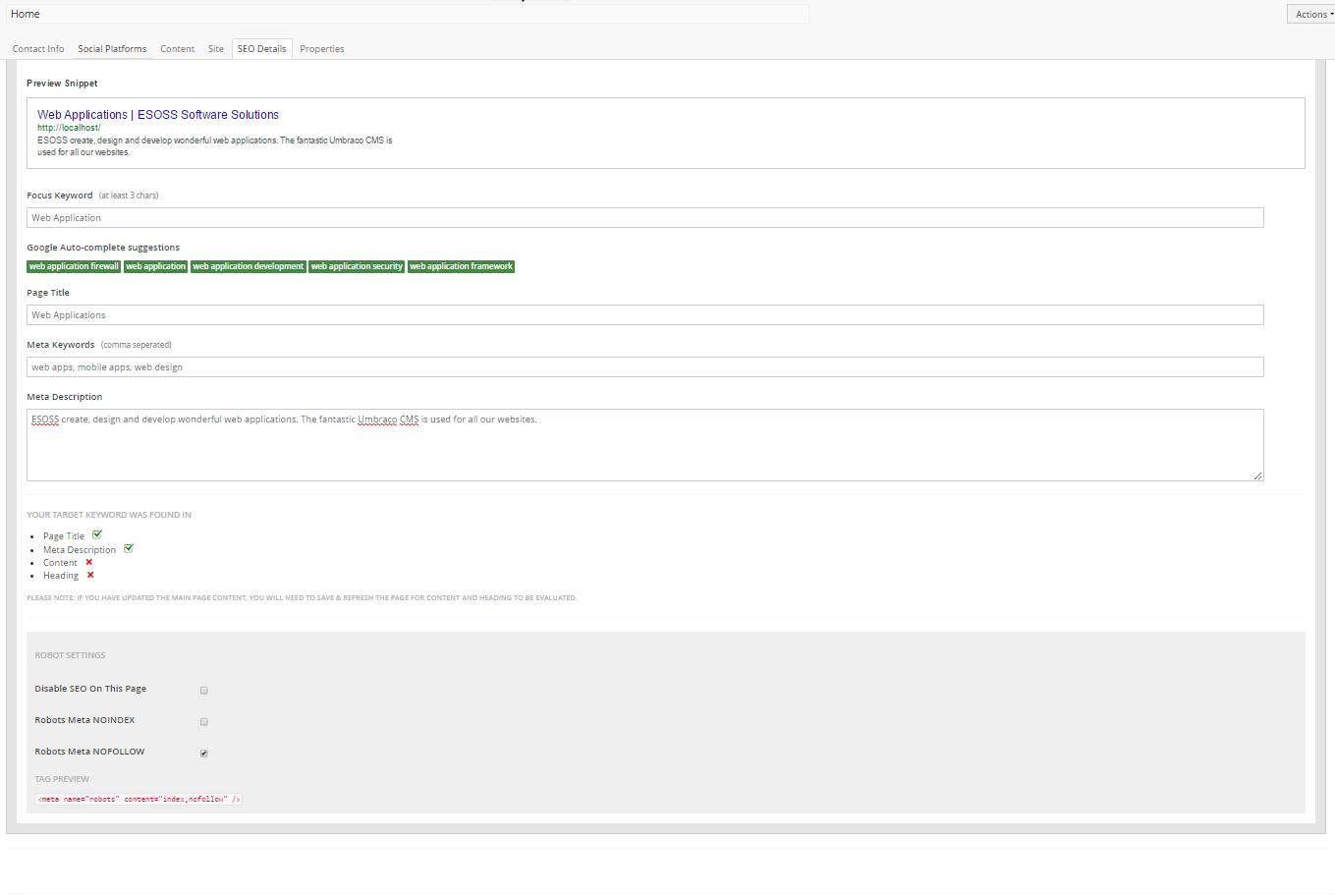The image depicts a website interface with various elements and sections:

At the top left-hand corner, there is a gray banner displaying the word "Home." To the right of the banner, there is a small rectangle, which appears to be labeled "Actions," though the text is somewhat difficult to discern due to its size.

Below the "Home" label on the left side, there is a vertical list of navigation links. The first one reads "Contact Info," followed by "Social Platforms," and then a third link which is partially obscured but might say "Common." Among these, one link is highlighted in white. Further down, beneath these navigation links, unbolded information is displayed, leading to another rectangular section labeled "Web Applications," highlighted in blue.

Below "Web Applications," there is a section with the text "ESO SS Software Solutions." Directly under this text is an area designated for a keyword input, evident from a lone rectangular box labeled "Keyword."

To the right, there are a series of five green highlighted rectangles, arranged in a grid. Following this grid, there is a text box for a "Page Title" and another section for "Keywords." 

Finally, there is an area labeled for a description with a long text box, containing a sentence with portions of its text underlined in red at the beginning and near the end. Below this, bullet points provide additional information. The bottom of the image features a gray banner with three lines of information paired with icons aligned to the right.